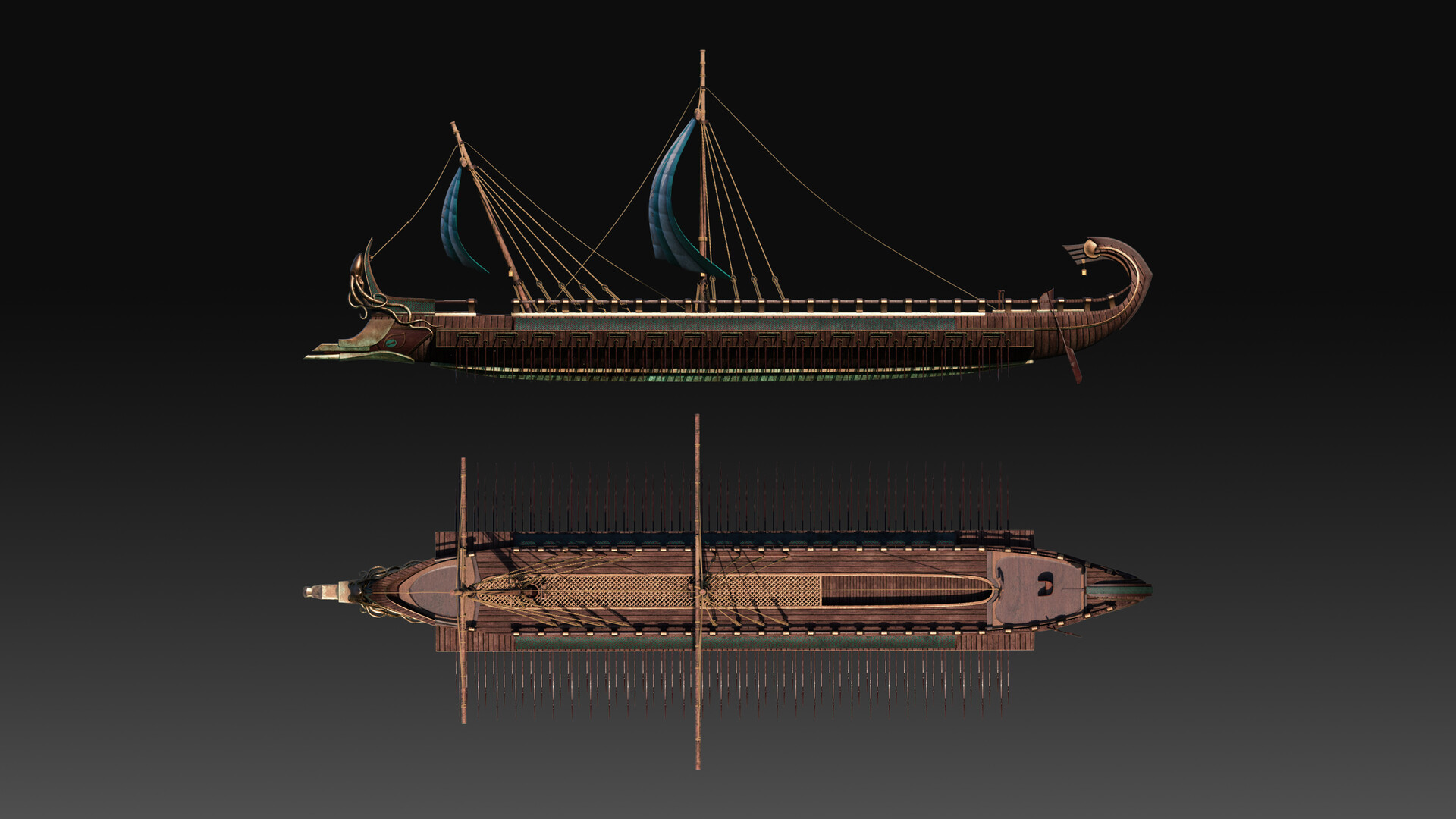The image depicts a meticulously crafted model of an ancient longboat, possibly a Viking ship, shown from two perspectives against a stark black background. The upper part of the image displays a side view of the ship, highlighting its wooden structure, long and thin form, and ornate details. The ship features a curved bow and stern resembling a serpent’s tail and possibly a dragon’s head. It has two brown masts with blue sails, and numerous ropes extending from vertical posts beside the sails. A silver horizontal line adorns the upper part of the hull with a decorative design beneath it, transitioning to a green bottom.

The lower part of the image offers a top-down perspective, revealing the ship's intricate rigging and width relative to its hull. This view showcases the vessel's rows of oars protruding from the sides, suggesting manual propulsion as well as sail power. The craftsmanship of the wooden model is evident in its detailed construction, including carved elements that could be interpreted as marine creatures such as dragons or octopuses. The background hues of dark blue and gray enhance the visibility of the model's elaborate features.